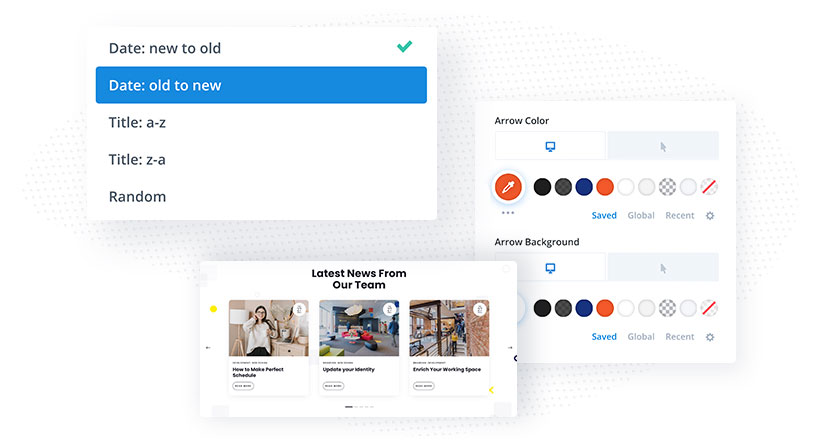This image showcases three distinct windows from a user interface on a website, presented against a gray gridded background.

The first window, located at the top-left, is a small rectangular filter sort interface. At the top of this window, there's an option labeled "Date: New to Old," marked with a green check mark. Directly beneath it is a blue-highlighted option that reads "Date: Old to New." The next options listed are "Title: A to Z," "Title: Z to A," and "Random."

Below this filter sort window, a prominent white window titled "Latest News From Our Team" displays three images. The first image depicts a woman standing in an office setting, wearing a sweater. The second image features a group of people seated in front of a TV or a similar screen. The third image on the right captures a scene of a city street.

Adjacent to, and partially behind the "Latest News From Our Team" window, there is a secondary window labeled "Arrow Color." This window displays a blue-colored image of a TV, accompanied by a grayed-out pointer to the right. It offers a variety of color options to choose from. Other elements within this window include options labeled "Save Global or Recent," "Arrow Background," and several mouse and color options for customization.

The detailed structure and content of these windows provide a comprehensive glimpse into the user interface and navigational elements of the website.